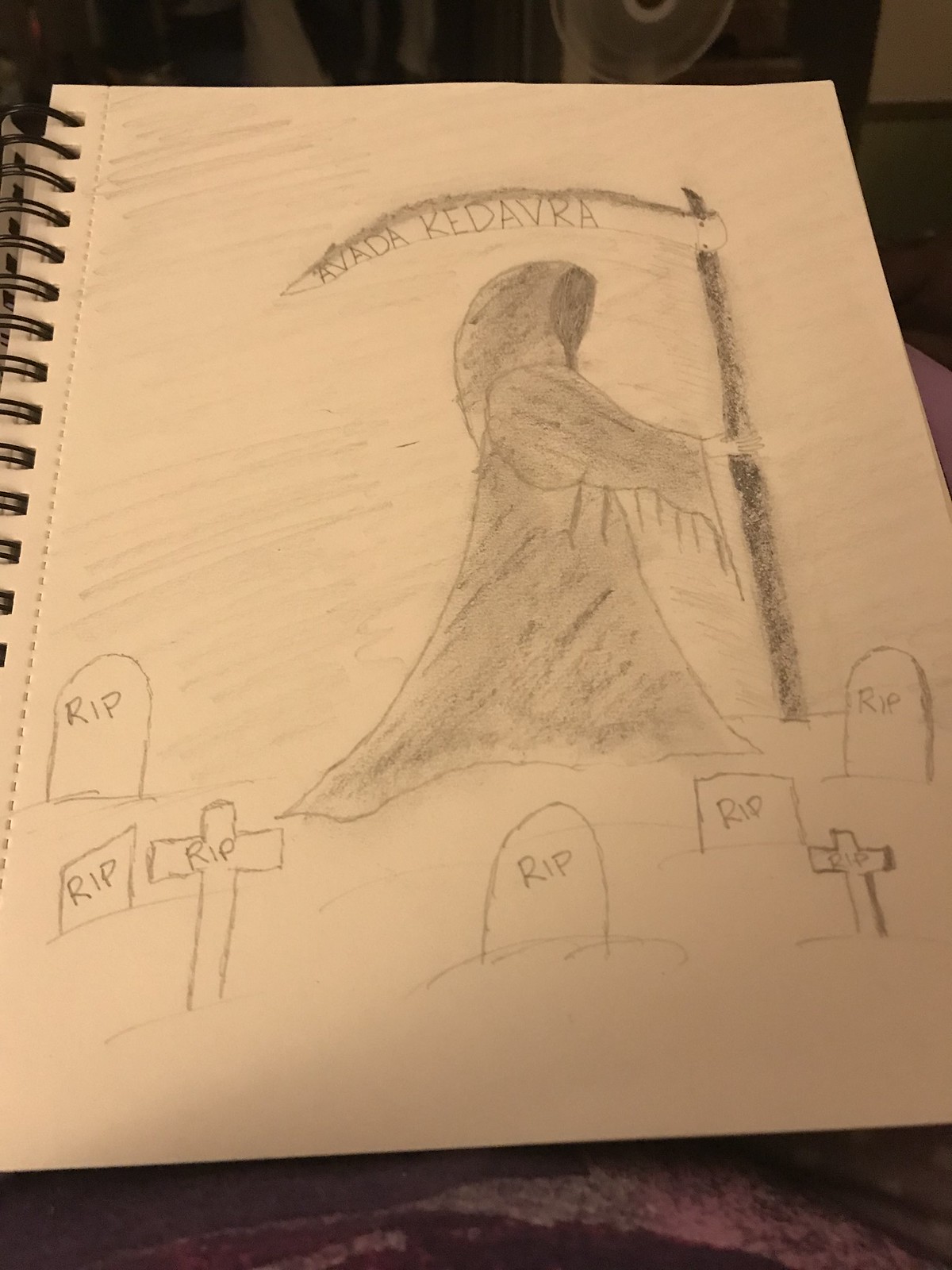In a detailed sketch within a spiral-bound notebook, ready for page removal via perforation, there is a haunting portrayal of the grim figure of Death. Death is captured in profile, adorned in an extensive, flowing dark robe, meticulously detailed with pencil marks to illustrate wrinkles. The robe’s generous fit is evidenced by its sagging sleeves, from which tattered fabric or tassels hang, revealing a skeletal right hand emerging thinly from the voluminous sleeve.

The robe's hood is drawn up, masking Death's face completely in dark shadow, an eerie void devoid of any features. Grasped in its right hand is the upright handle of a foreboding scythe. Inscribed on the blade is the phrase "Avada Kedavra," a chilling nod to the Harry Potter series' infamous killing curse.

Death strides through an ominous graveyard dotted with various headstones. The scene includes two cross-shaped headstones, two rectangular ones, and three taller stones with rounded tops, each bearing the inscription "R.I.P.", symbolizing "rest in peace."